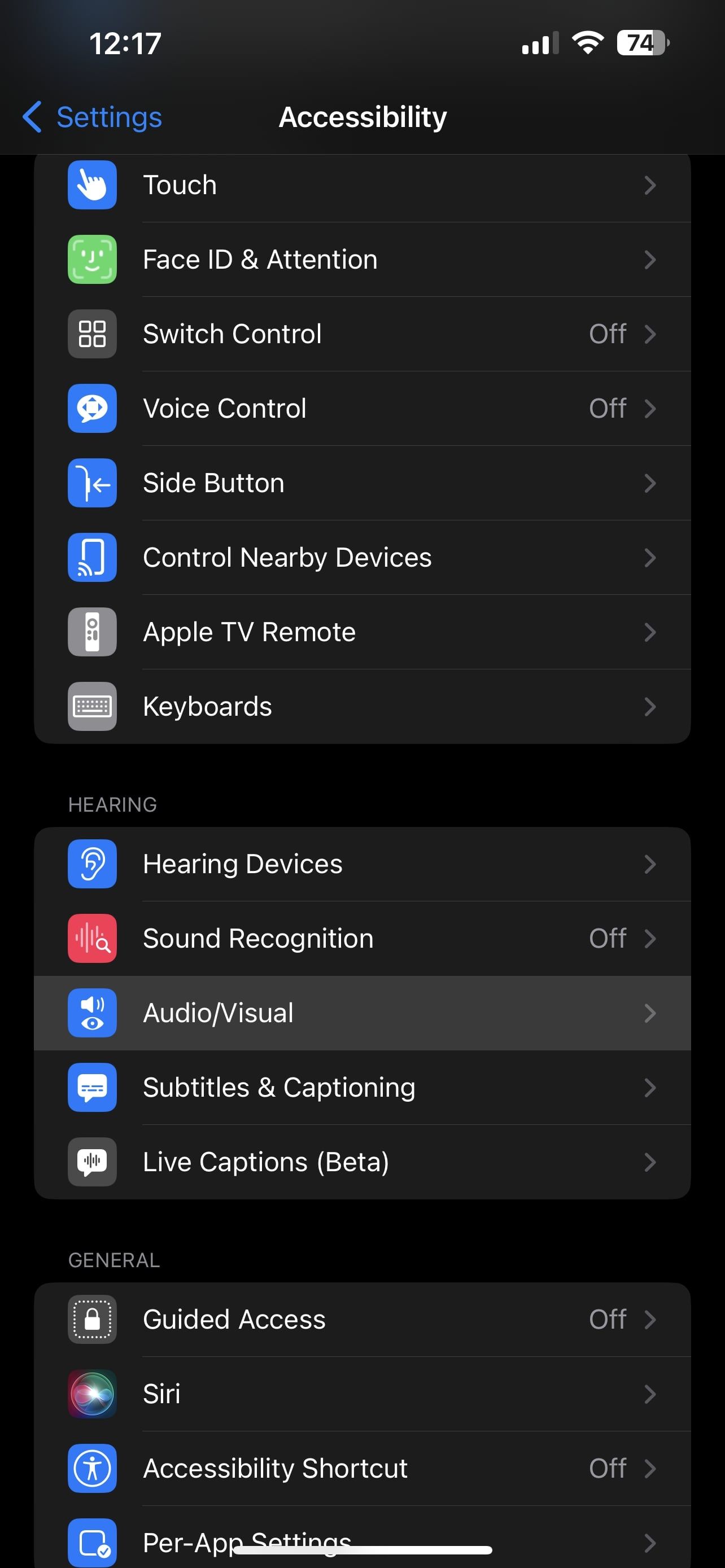A detailed screenshot captured in portrait orientation from a smartphone on a day at 12:17 PM. The image is in color with the phone displaying three out of four bars of signal reception and a battery level at 74%. The screenshot mainly showcases the accessibility settings menu, accessed via Settings > Accessibility. The visible sections include options for Touch, Face ID and Attention, Switch Control, Voice Control, Side Button, Control Nearby Devices, Apple TV Remote, and Keyboards. Beside each of these options, there are arrows indicating further configurable settings. In the Hearing section, options for Hearing Devices, Sound Recognition (currently off), Audio/Visual, Subtitles & Captioning, and Live Captions (Beta) are displayed. Below the Hearing section, but not fully visible without scrolling further, are additional settings like Guided Access (off), Siri, Accessibility Shortcut (off), and Per App Settings. The interface features a primarily black background with white text for clarity.